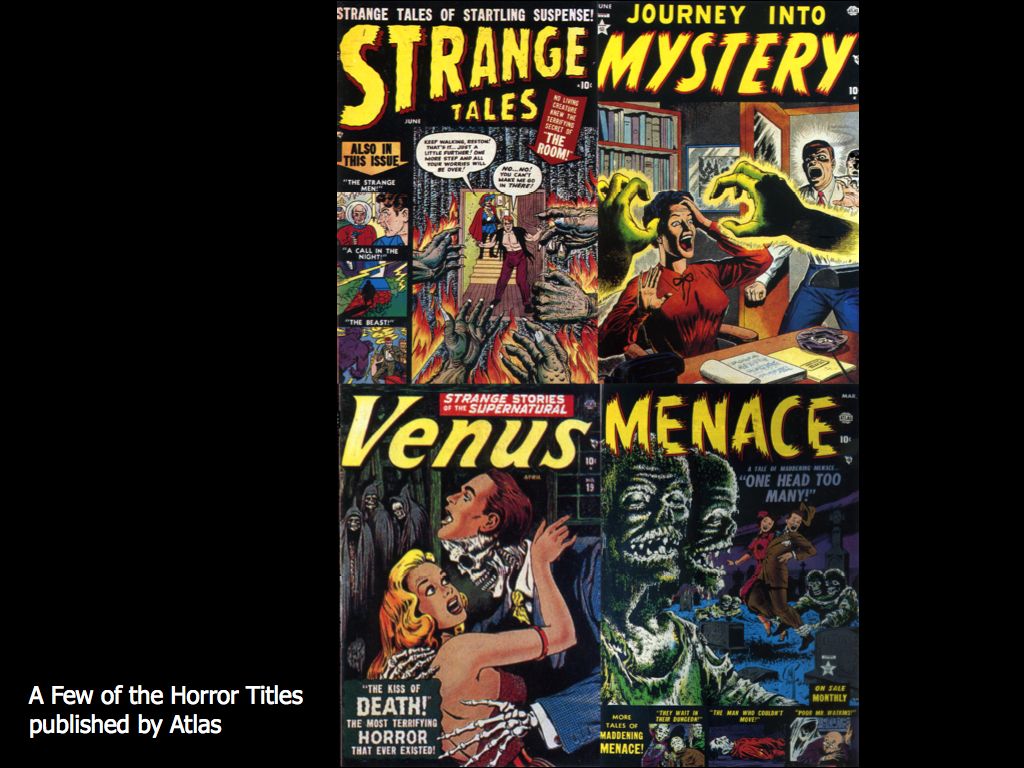The image showcases four vintage comic book covers, displayed against a black background, highlighting the intricate and colorful artwork typical of mid-20th century horror comics. Each cover is steeped in hues of red, blue, yellow, black, gray, and white, depicting scenes filled with zombies, skeletons, ghosts, and terrified humans, mostly women. 

On the top left, the cover reads "Strange Tales of Startling Suspense," with "Strange Tales" boldly written in yellow. Opposite this, on the top right, another cover reads "Journey into Mystery," also highlighted in bold yellow letters. 

The bottom left features "Strange Stories of the Supernatural: Venus, the Kiss of Death," with "Venus" prominently displayed in bold yellow, and the background punctuated by chilling descriptions of horror. Finally, the bottom right cover reads "Menace: One Head Too Many," with "Menace" emblazoned in bold yellow capital letters.

The left border includes the inscription, "A few of the horror titles published by Atlas," in white letters, hinting at the publisher's legacy in the horror genre. The overall composition emphasizes the dramatic and suspenseful nature of these classic comic book covers.